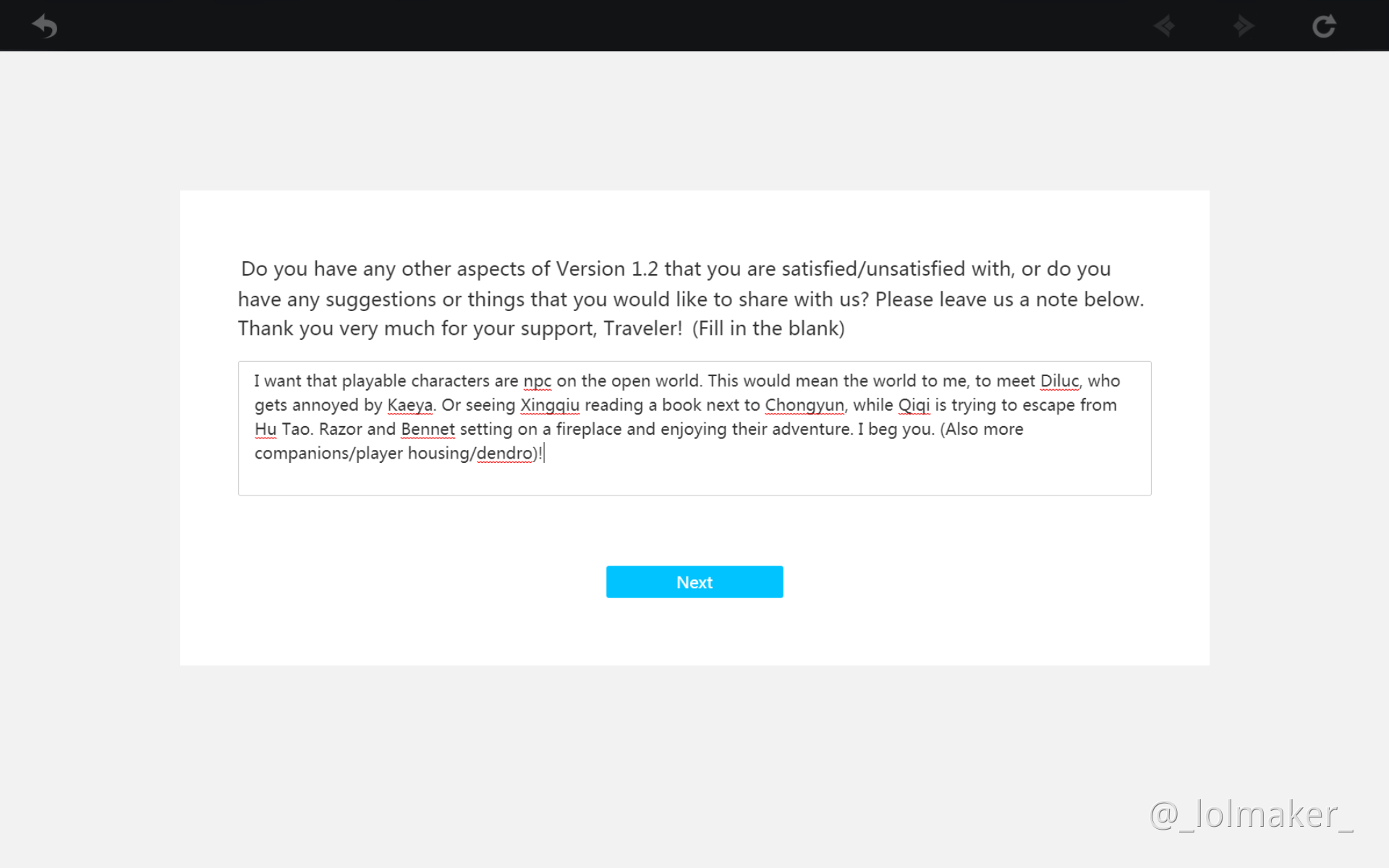This screenshot displays a user interface with a predominantly gray background. At the top, there's a black tab containing a back button and a refresh button. Centrally located on the gray background is a white text box. Inside this text box, the following message is displayed:

"Do you have any other aspects of version 1.2 that you are satisfied/unsatisfied with? Or do you have any suggestions or things that you would like to share with us? Please leave us a note below. Thank you very much for your support, traveler. (Fill in the blank)."

A user's response is displayed below the prompt, stating:

"I want that playable characters are NPC in the open world. This would mean the world to me. To me, seeing Diluc get annoyed by Kaeya, or Xingqiu reading a book next to Chongyun while Qiqi is trying to escape from Hu Tao, Razor and Bennett sitting by a fireplace and enjoying their adventure. I beg you. (Also more companions/player housing/dendro!)"

Notably, certain words in the user's response, such as "NPC," "Diluc," "Kaeya," "Xingqiu," "Chongyun," "Qiqi," "Hu," "Bennett," and "dendro," are underlined in red, presumably indicating spelling errors or unrecognized terms by the computer's spell-check.